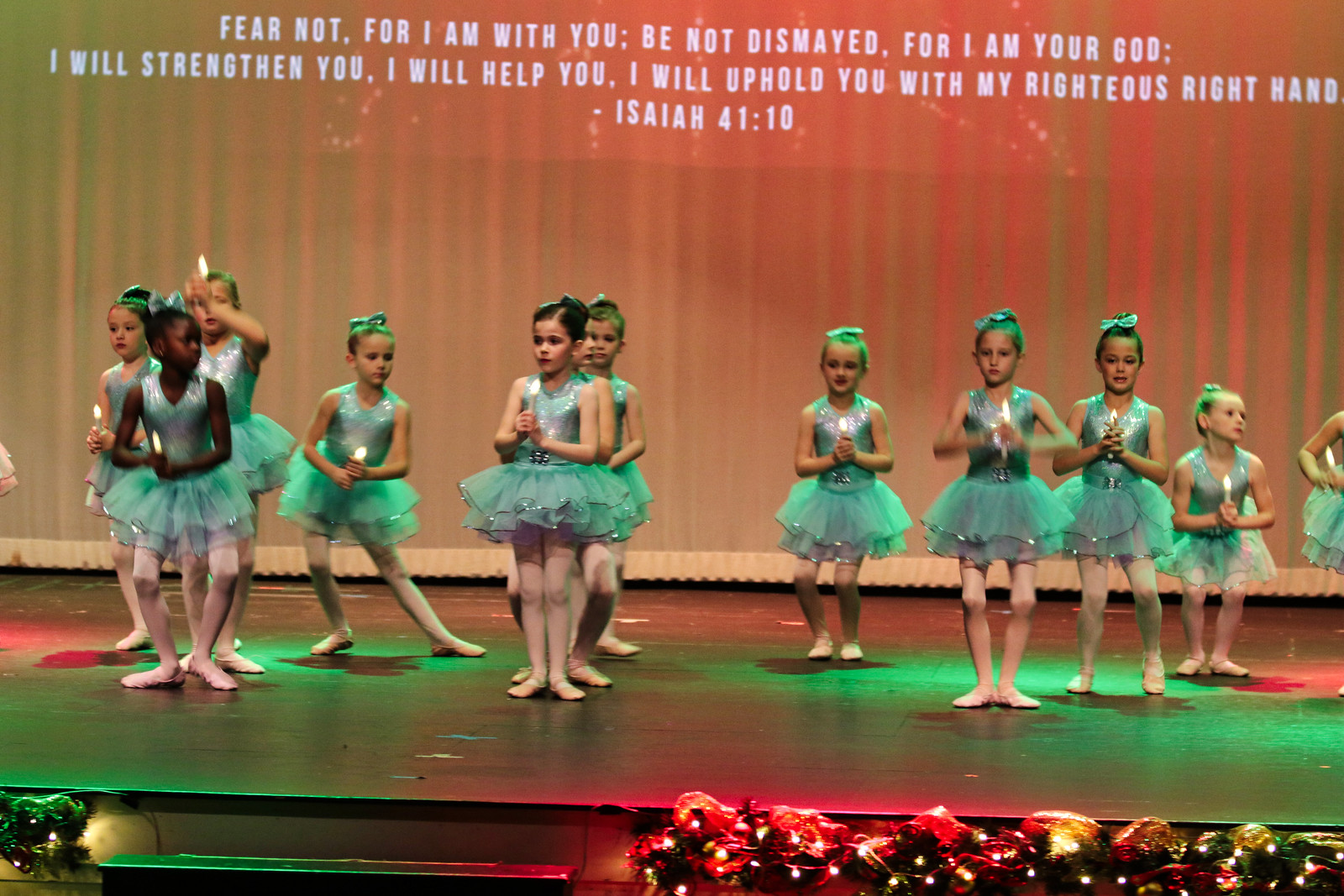This photograph captures a heartwarming scene of approximately ten young girls performing a dance recital on a festively decorated stage. The stage backdrop features an orange curtain with a prominently displayed Biblical quote from Isaiah 41:10 in white font: "Fear not, for I am with you; be not dismayed, for I am your God. I will strengthen you, I will help you, I will uphold you with my righteous right hand." The stage is adorned with green, red, and yellow Christmas lights and garland, adding to the holiday spirit. The girls, all dressed in light green ballerina tutus, are holding candles and performing ballet moves, including pliés with their knees bent slightly and toes pointed outward, hands in prayer positions. Some of the dancers are looking directly at the camera, while others gaze to the sides, capturing a blend of concentration and innocence. The overall ambiance and the festive decorations suggest this event is a Christmas-themed performance, emphasizing the season's joyous and spiritual message.